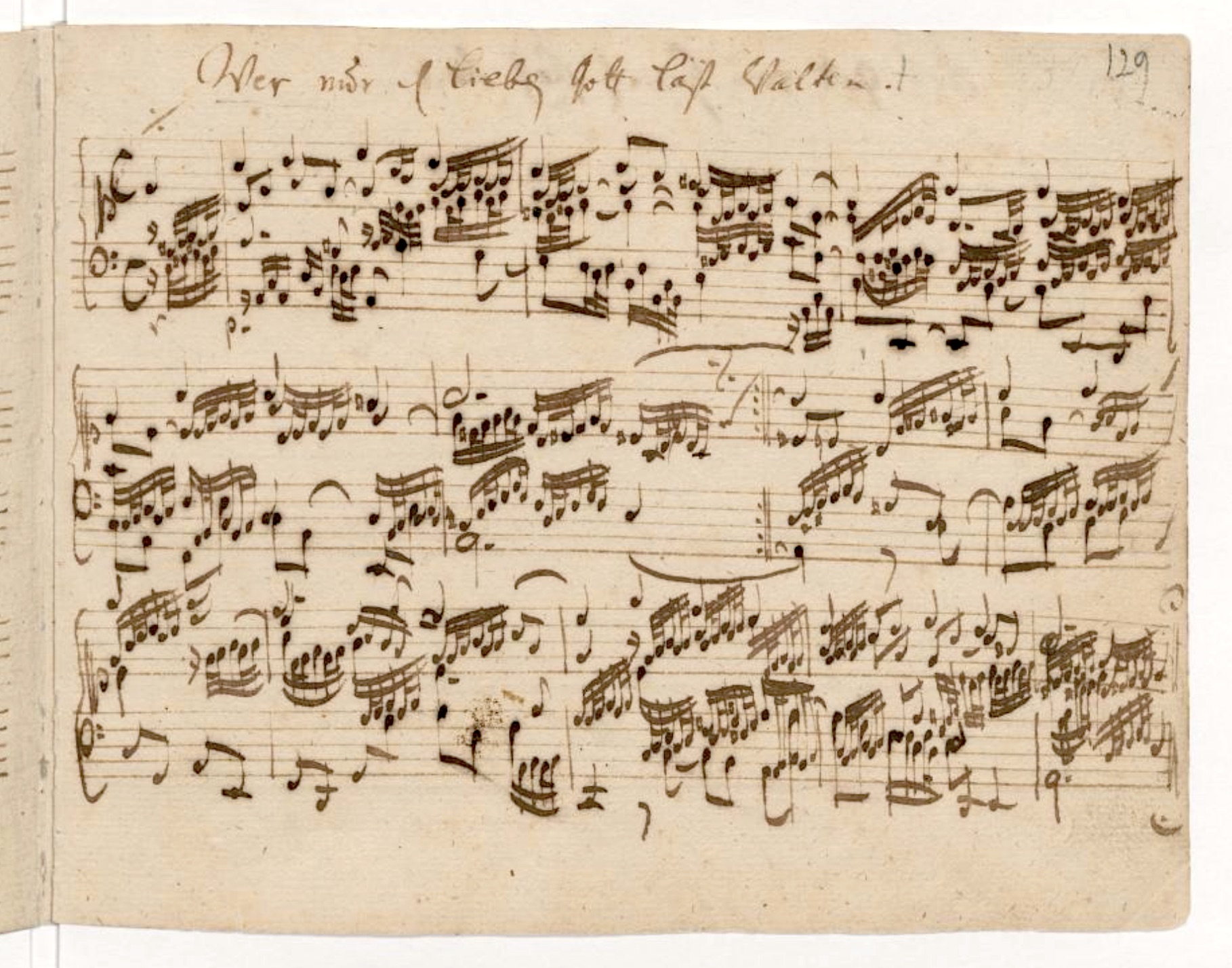This image depicts an old, horizontal rectangular sheet of music, showing significant wear and tear with a faded brown coloration that hints at its vintage nature. The page is part of a larger book or notebook, evident from the visible binding ridge along the left edge, as well as the cut-off end of another page peeking from the left side. The title of the piece, written in cursive at the top, is difficult to decipher, possibly in a foreign language, which seems to be either German or another Latin-based script. A notable detail is the number "129" penned in the top right corner, marking this as page 129 of the volume. The sheet features three horizontal rows of musical staves, with each stave containing five lines filled with numerous handwritten musical notes, signifying a possibly complex musical composition.